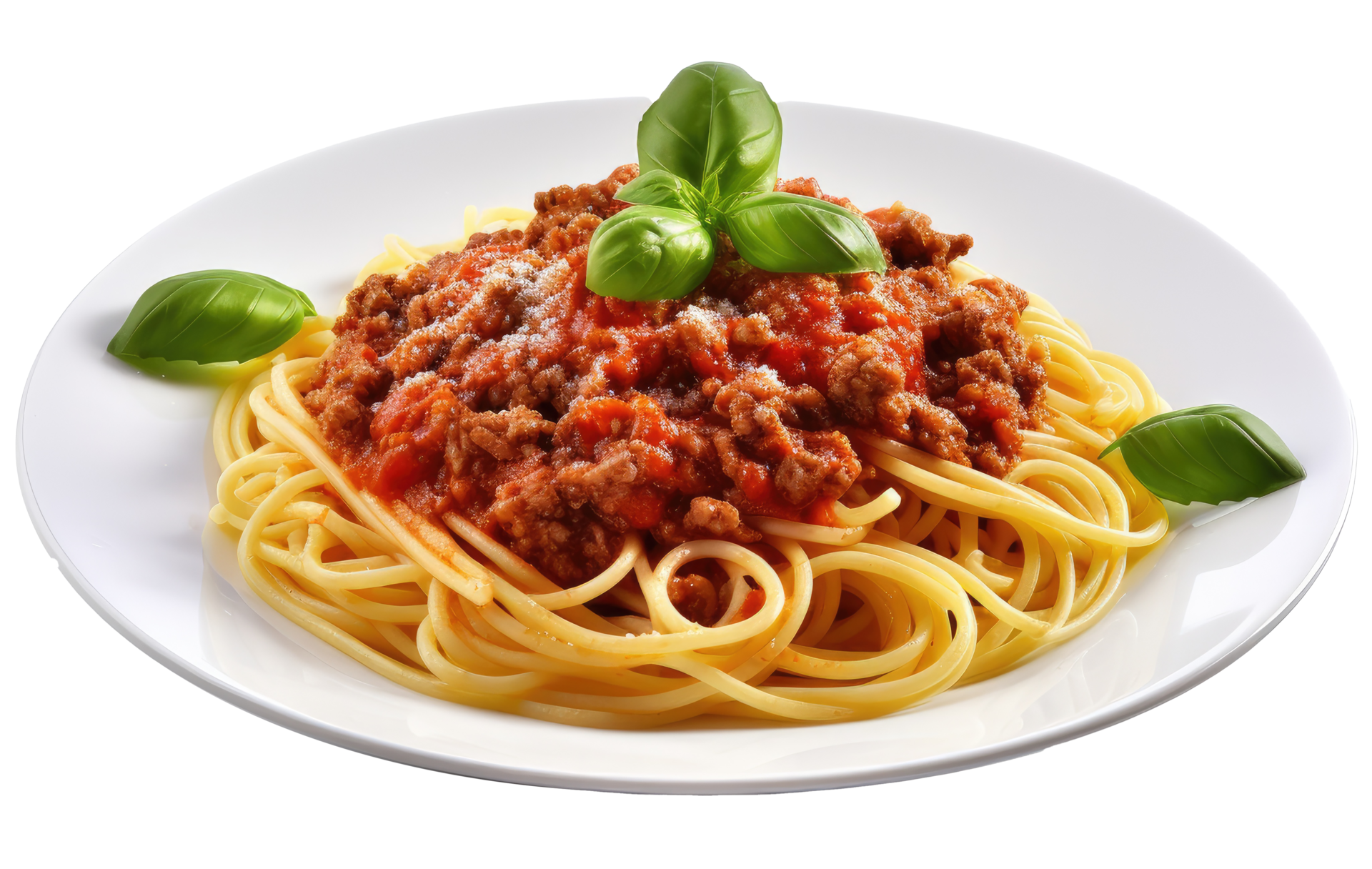This detailed photo showcases a round white plate set against an all-white background. At the base of the plate lies a generous serving of yellowish noodles, resembling spaghetti or macaroni. These noodles are topped with a hearty meat sauce, predominantly red from the tomato chunks interspersed with brown bits of hamburger meat. The sauce is spread liberally over most of the noodles. Adding a touch of freshness and color, three to four green leaves are clustered together at the top of the dish, while additional single green leaves adorn the upper left and right sides of the plate. Slightly hidden beneath the green leaves at the very top and scattered over the red meat sauce is a sprinkling of white Parmesan cheese, adding a final garnish to this appetizing presentation.